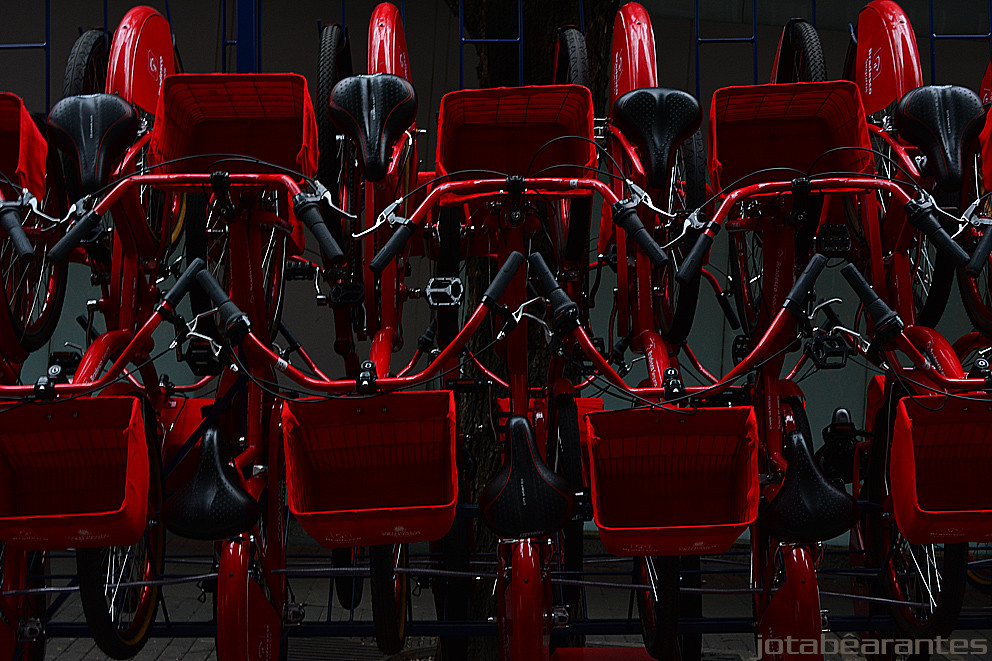This image features a striking display of bright apple-red bicycles neatly arranged on a black background, each bike meticulously hung on a dark blue rack. The bicycles are arrayed in two distinct rows, with four bicycles positioned on the upper level and another four on the lower level. Each bicycle is outfitted with a shiny black seat, clean black handlebars with black grips, and sleek silver handbrakes and pedals highlighted by silver accents. The standout detail of each bike is the vivid red wire baskets, complemented by red metal frames and handlebars adorned with silver stripes for a high-end appearance. Adding to the race car-like allure, there are small front wheel guards featuring a symbol on the side. The bottom right corner of the photo is marked with the name "Jada Bear Barenties" displayed in a translucent white font. The overall composition is dynamic, showcasing the bicycles' craftsmanship and vibrant colors against the stark contrast of the background.